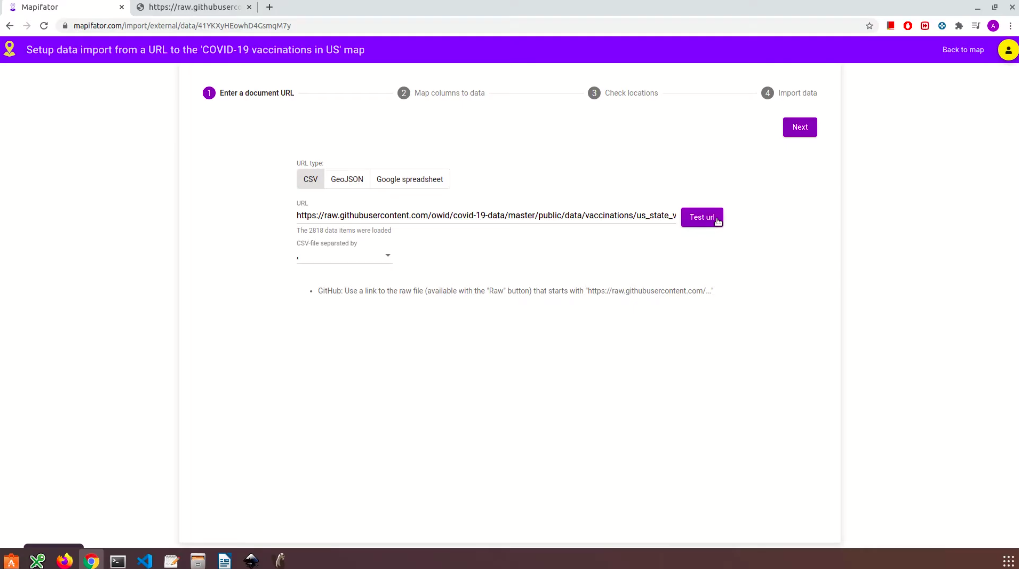The screenshot showcases a Mac desktop displaying a webpage with a primarily white background and substantial blank space, making it hard to discern detailed content. At the top of the page, a bright purple header includes a URL that vaguely resembles "mapfinder.com" or something similar. The webpage appears to be related to setting up a data import for a COVID-19 vaccinations map in the US.

On the left side of the page, there is a yellow location option, and on the right side, there is a potential sign-in or account button. Below the header, the webpage instructs users to "Enter a dissemination URL" as part of Step 1. This section includes a field where a URL from raw GitHub user content has already been entered.

Further down, navigation options suggest different types of data formats available for import, including CSV, GeoJSON, and Google Spreadsheets. Each format option is organized in a tab-like setup, with the current view likely set to CSV. A "Test URL" button is visible, suggesting the ability to verify the entered URL before proceeding to the next step.

Additionally, at the top of the browser, there is another open tab, though its contents are not identifiable from the screenshot.